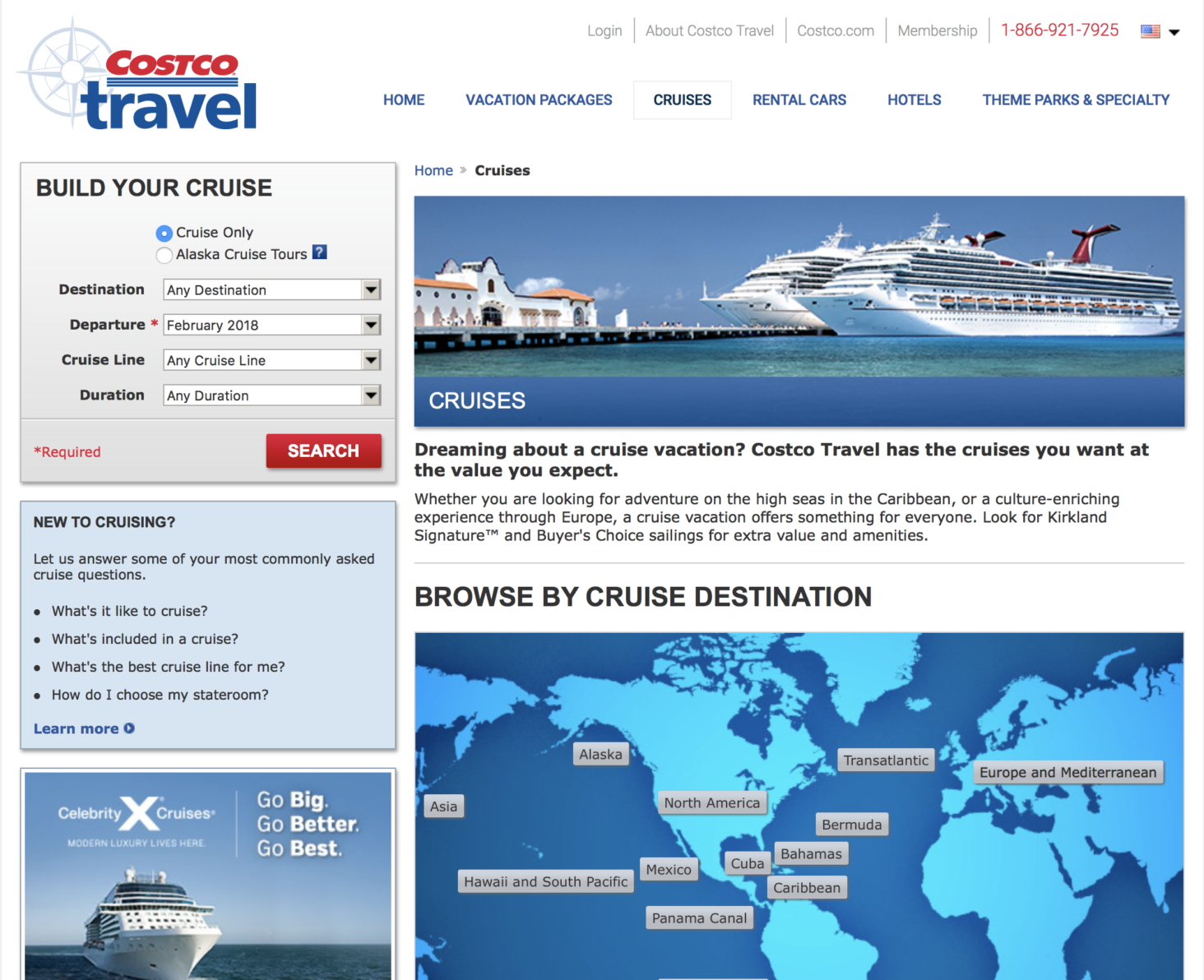Explore the world with Costco Travel! From vacation packages and cruises to rental cars, hotels, and theme parks, Costco Travel offers a variety of travel options to suit your needs. Whether you’re dreaming of an adventure on the high seas in the Caribbean or a culturally enriching experience through Europe, Costco Travel has the cruise vacations you desire at the value you expect. Learn about membership benefits, browse destination options, and get answers to your cruising questions. Contact Costco Travel at 1-866-921-7925 for assistance and start planning your next journey today.